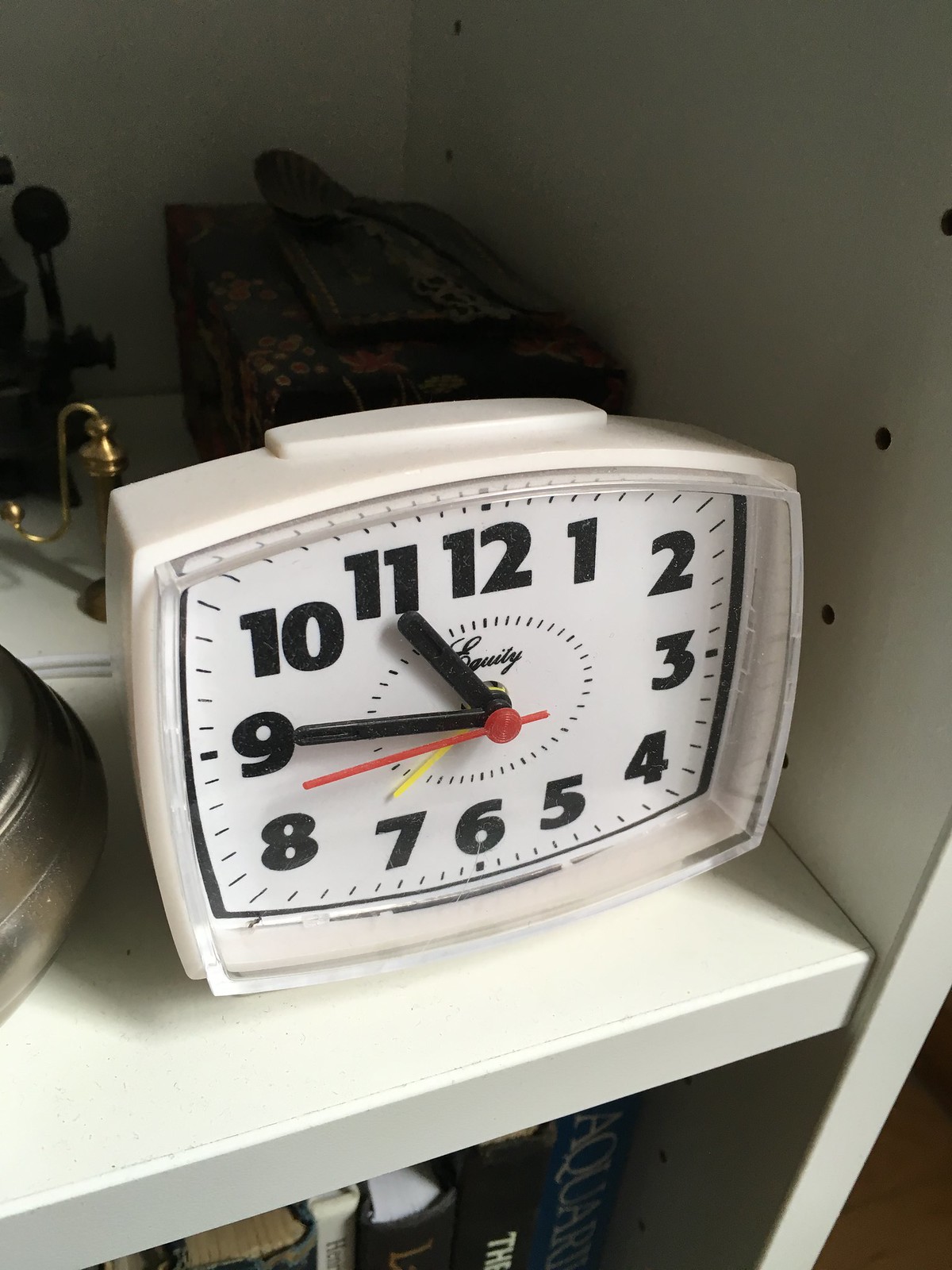The image depicts a small, white, do-it-yourself wooden stand with a clock prominently displayed on the top shelf. The clock, which features a rectangular white plastic body, has a white face with black hands for the hours and minutes, a red second hand, and a yellow hand for the alarm. The numbers 1 through 12 are printed in black, and the brand name, "Equity," is partially visible in cursive. The current time on the clock is approximately 10:45, with the alarm set for 7:30. Behind the clock, there's a small black box decorated with flowers and what appears to be an antique-looking spoon. An item resembling an antique phone is partially visible. The bottom shelf of the stand holds a collection of hardcover books, one of which seems to start with "Aqua," likely referring to "Aquarium."